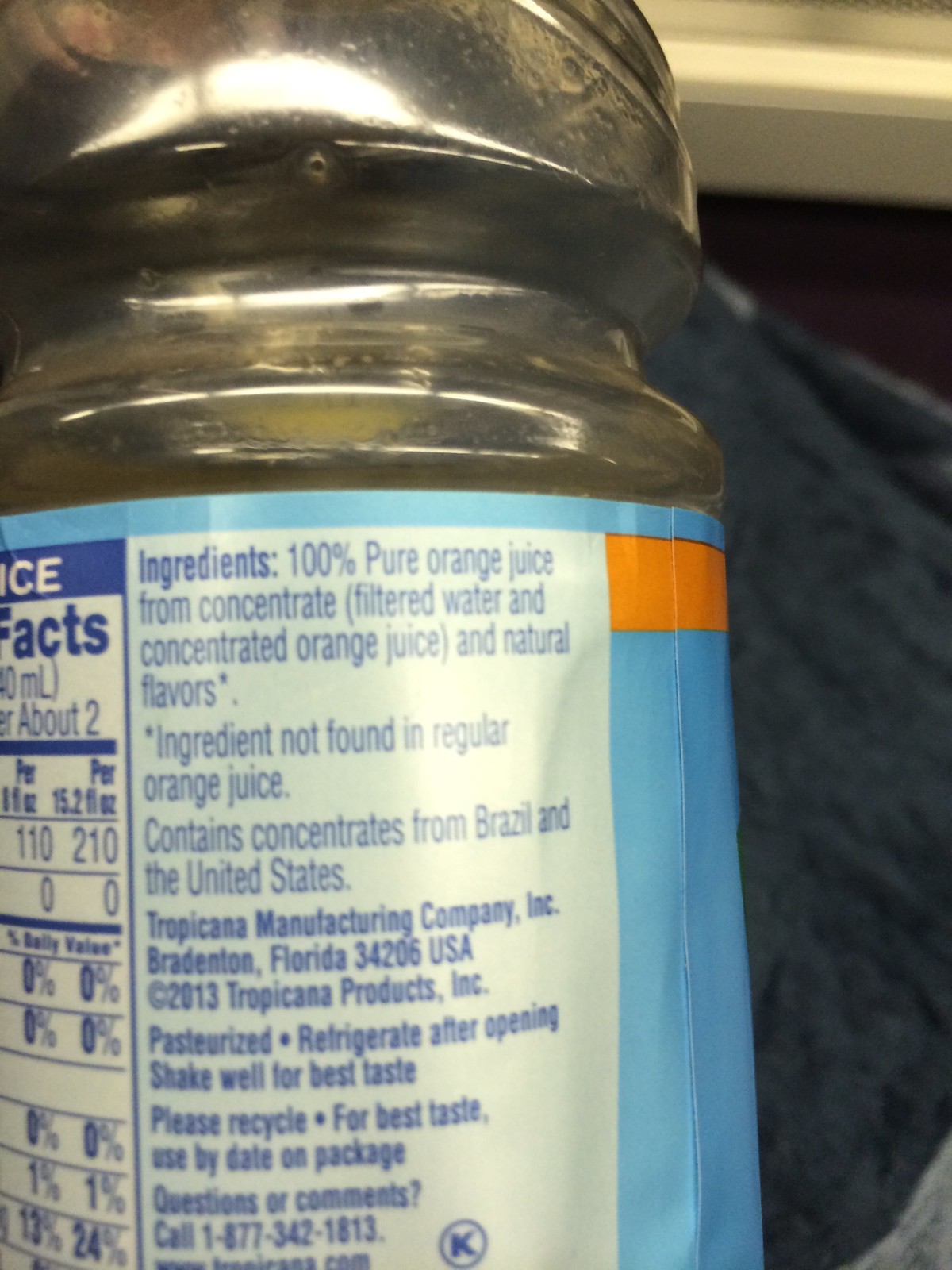The image depicts a clear plastic bottle adorned with a light teal or light blue plastic wrapper. The wrapper features prominent sections such as the nutrition facts block and a partially visible ingredients column. Additional information includes the manufacturer's details and location, along with various instructions: "Pasteurize," "Refrigerate after opening," "Shake well for best taste," "Please recycle," and "For best taste, use by the date on package." There's also a prompt for questions or comments, directing the viewer to call a provided phone number. Toward the upper right of the wrapper, there's a darker orange bar. The background of the image appears to show a dark gray or perhaps black cloth to the right of the bottle, and a white item with noticeable light reflections, contributing to the overall composition.